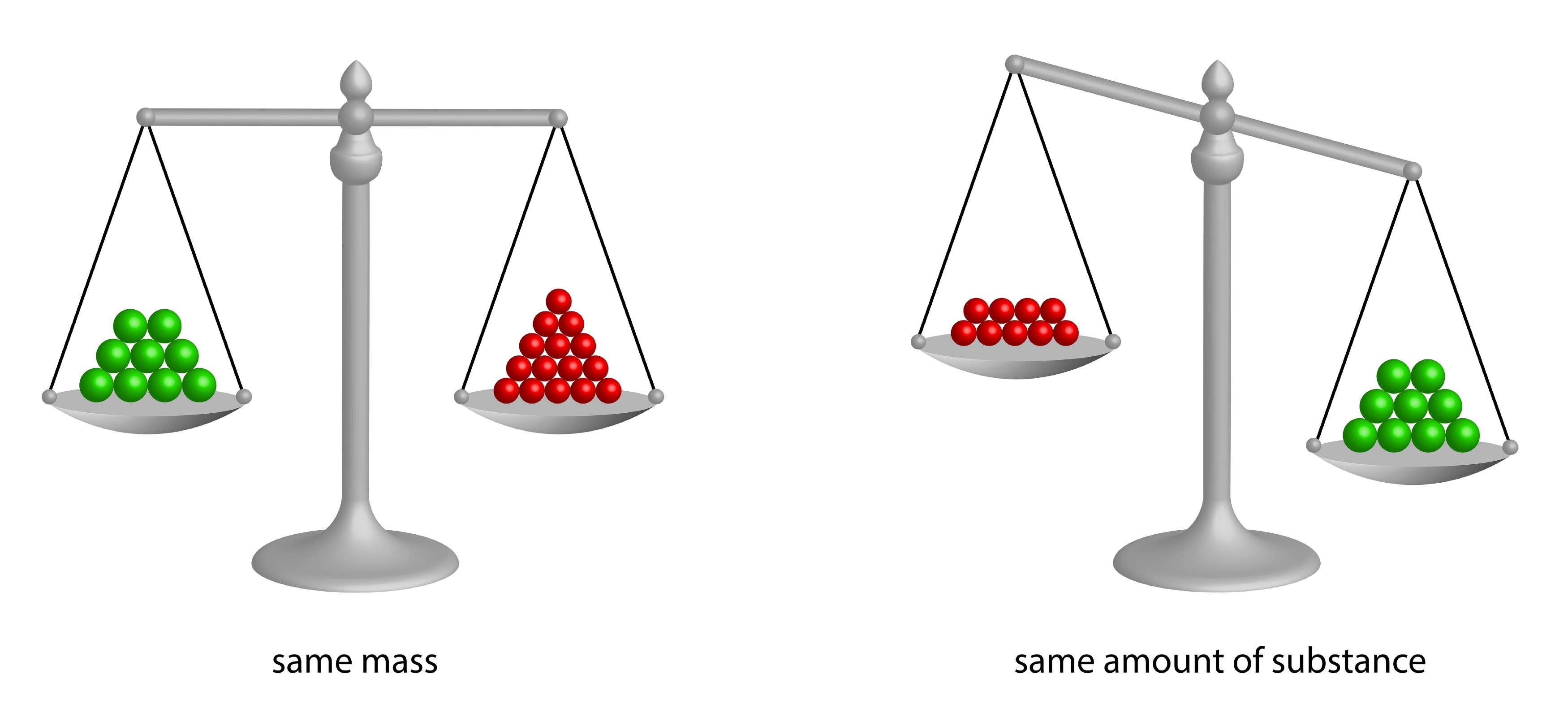This is a digitally rendered scientific diagram from a textbook, featuring two balance scales illustrating different concepts of mass and substance. In the first image, the scale shows an equal balance with the caption "same mass." On the left pan, there are ten large green balls stacked evenly, while on the right pan, there are fifteen smaller red balls. This depiction demonstrates that although the number of balls differs, the total mass remains equal. In the second image, the scale is titled "same amount of substance" and reveals an imbalance, tilting downward to the right. Both pans hold an equal number of balls — nine green balls on the right and nine smaller red balls on the left. This indicates that despite having the same number of items (substance), the green balls are heavier than the red balls, leading to an uneven distribution of weight. Each scale visually represents distinctions between mass and quantity, clarifying that identical amounts of substance do not always equate to similar masses.